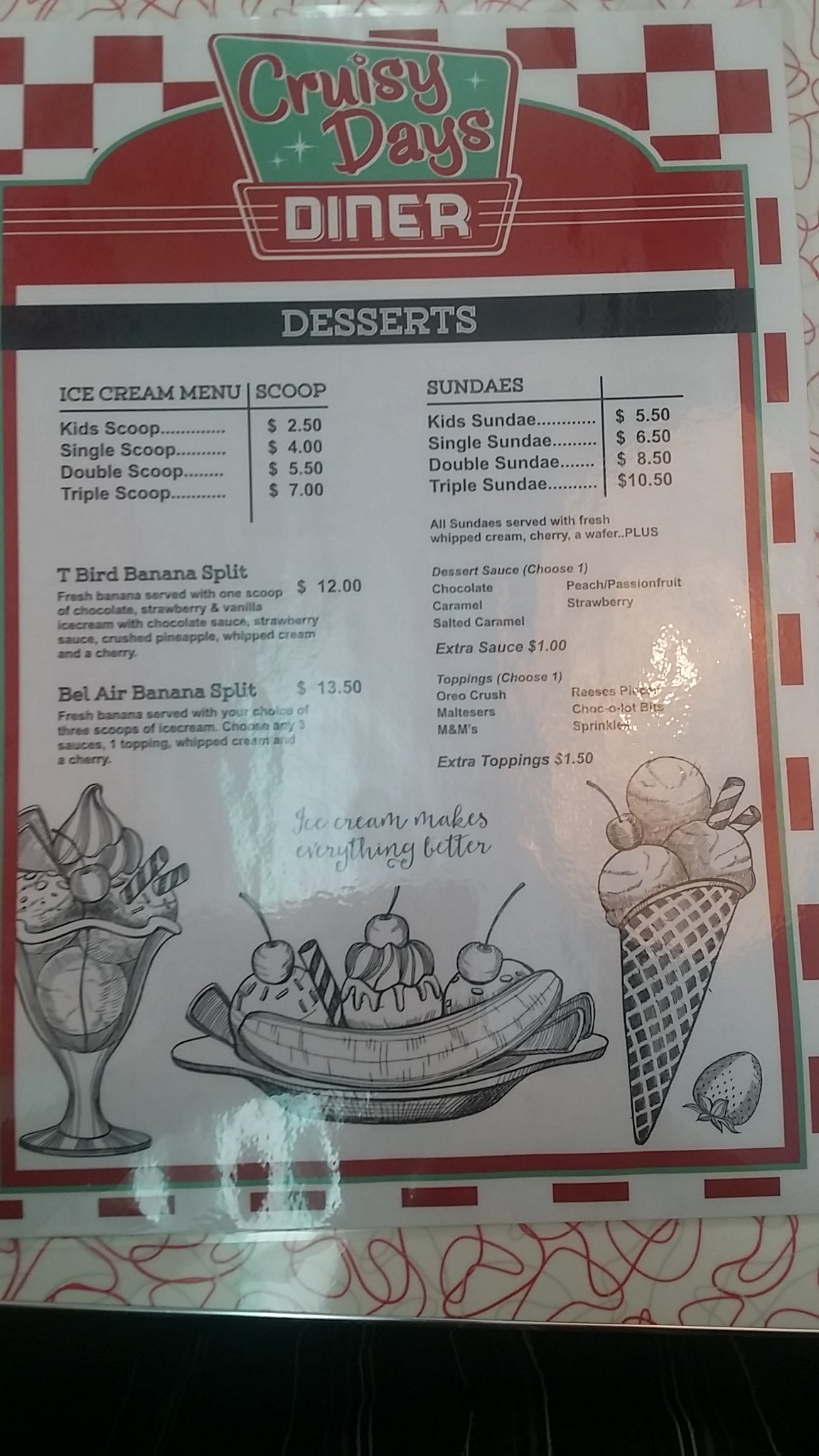This photograph captures a dessert menu placed on a restaurant tabletop. The tabletop features a white background adorned with red squiggle lines, adding a playful touch to the scene. The menu itself exudes a charming retro vibe with its red and white checkered design, framed by a red border that prominently displays the "Cruisy Days Diner" logo – reminiscent of classic diner signage.

Dominating the top of the menu is a black banner with "Desserts" written in bold white letters, immediately drawing the reader's attention. Below this, the menu offers an array of delectable ice cream choices. There are multiple scoop options in varying sizes, alongside an enticing selection of sundaes. Notably, the menu lists the "T-Bird Banana Split" and the "Bel Air Banana Split" as highlights among the dessert offerings. Though some details are difficult to discern, it is evident that there are various toppings and sauce options available to customize these treats.

At the bottom of the menu, a series of black and white sketch drawings beautifully illustrate the dessert selections. These include a detailed depiction of a banana split, a whimsical curve-handled pedestal glass holding a sundae, and a waffle cone with multiple scoops of ice cream.

Overall, this image not only showcases the menu but also captures the nostalgic essence of Cruisy Days Diner, making one yearn for a sweet, indulgent treat.